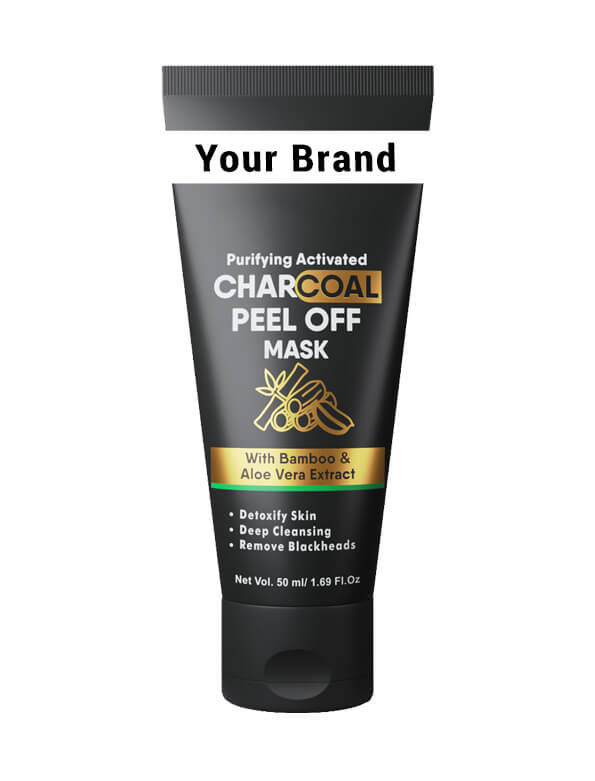The image showcases a sleek and masculine black tube designed for a charcoal peel-off mask, standing upright on its black cap. At the top of the tube, a white band is reserved for branding purposes, displaying "your brand" in black letters. Below this, the product description is prominently featured in white text, reading "charcoal peel-off mask." A gold symbol resembling rolls is positioned beneath the description.

Following this, a gold banner with black text highlights the key ingredients: "with bamboo and aloe vera extracts." Under the banner, three bullet points in white lettering detail the mask's benefits: "detoxify skin," "deep cleansing," and "remove blackheads." The net volume of the product is clearly stated at the bottom in fine white print: "net volume 50 ml / 1.69 fl oz." The overall design and detailed annotations make it suitable for marketing purposes, such as on an eBay listing.